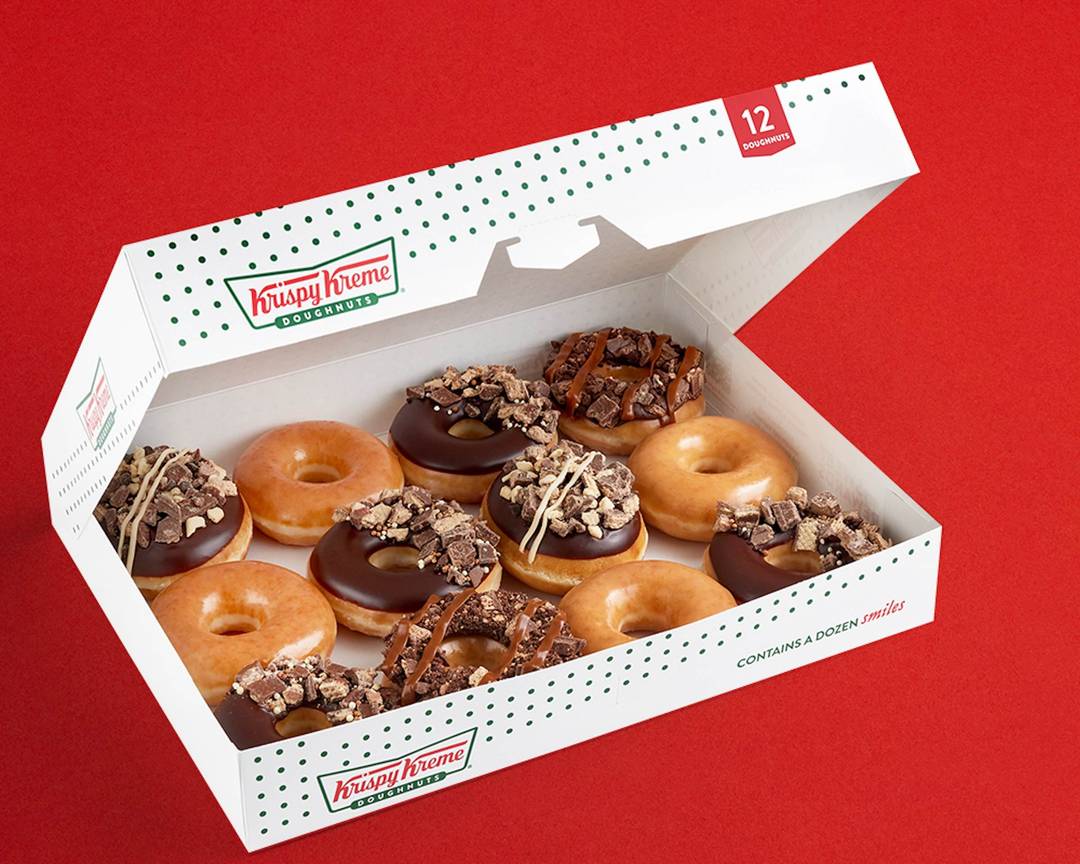The image showcases an open, rectangular white Krispy Kreme box, slightly folded like a pizza box and tilted counterclockwise at about a 20-degree angle. The box, adorned with Krispy Kreme's polka dot design, prominently displays the phrase "Contains a dozen smiles" in red text along the front. Positioned against a very bright red background, the box is filled with an assortment of 12 donuts arranged in a 4x3 grid. The variety includes classic glazed donuts, chocolate glazed donuts with possible caramel swirls, and chocolate donuts topped with what appears to be white chocolate and milk chocolate sprinkles. The box flap, open at a 45-degree angle, also features a sign that reads "twelve donuts," adding to the inviting presentation.